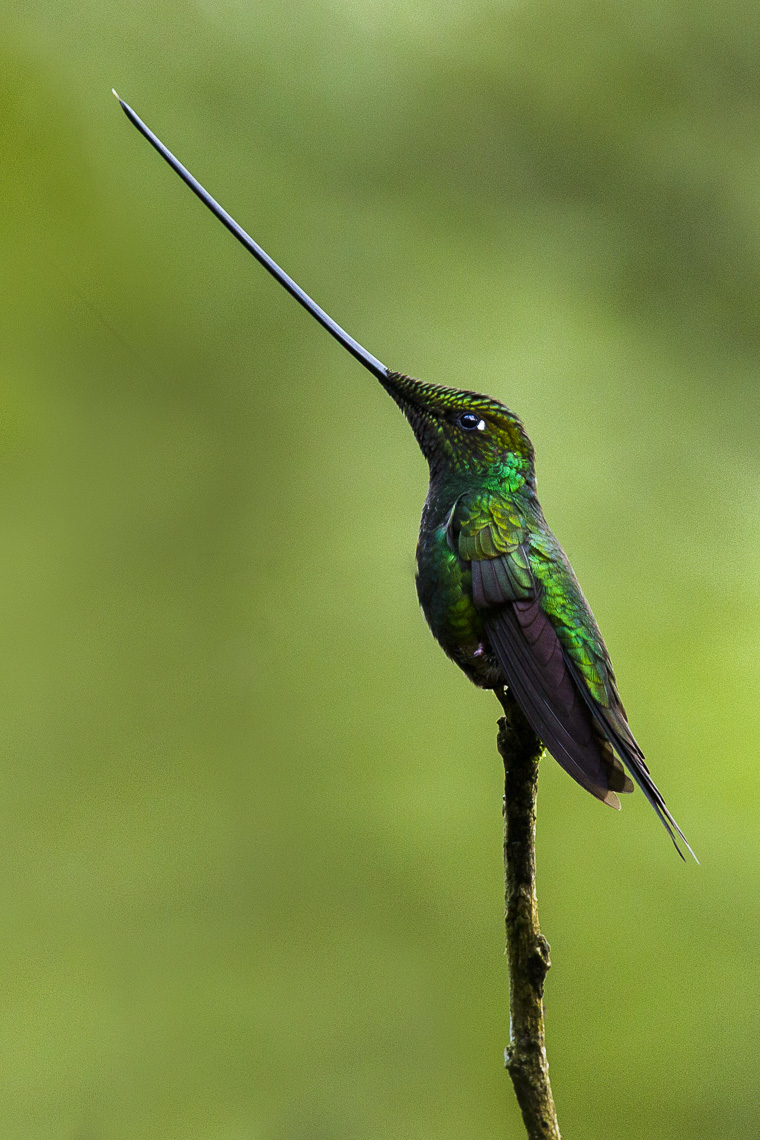This stunning close-up photograph captures a vibrant hummingbird in exquisite detail. The bird's elongated beak, reminiscent of a slender sword, hints at its adaptation for accessing nectar deep within flowers. The hummingbird's head is a mesmerizing dark purple, accented with iridescent green feathers that seamlessly blend into turquoise hues cascading down to its collar. The breast showcases a captivating spectrum of purplish indigo, interspersed with iridescent green and blue hues. The wings are a visual symphony, starting with a turquoise iridescence that shifts into a yellowish-green before culminating in a deep violet purple. The delicate, shimmering wings are a testament to the bird's intricate beauty. Adding to the composition, the hummingbird is perched gracefully on a stick. This photograph not only highlights the bird's vibrant colors but also its elegance and grace, making it a truly gorgeous capture.